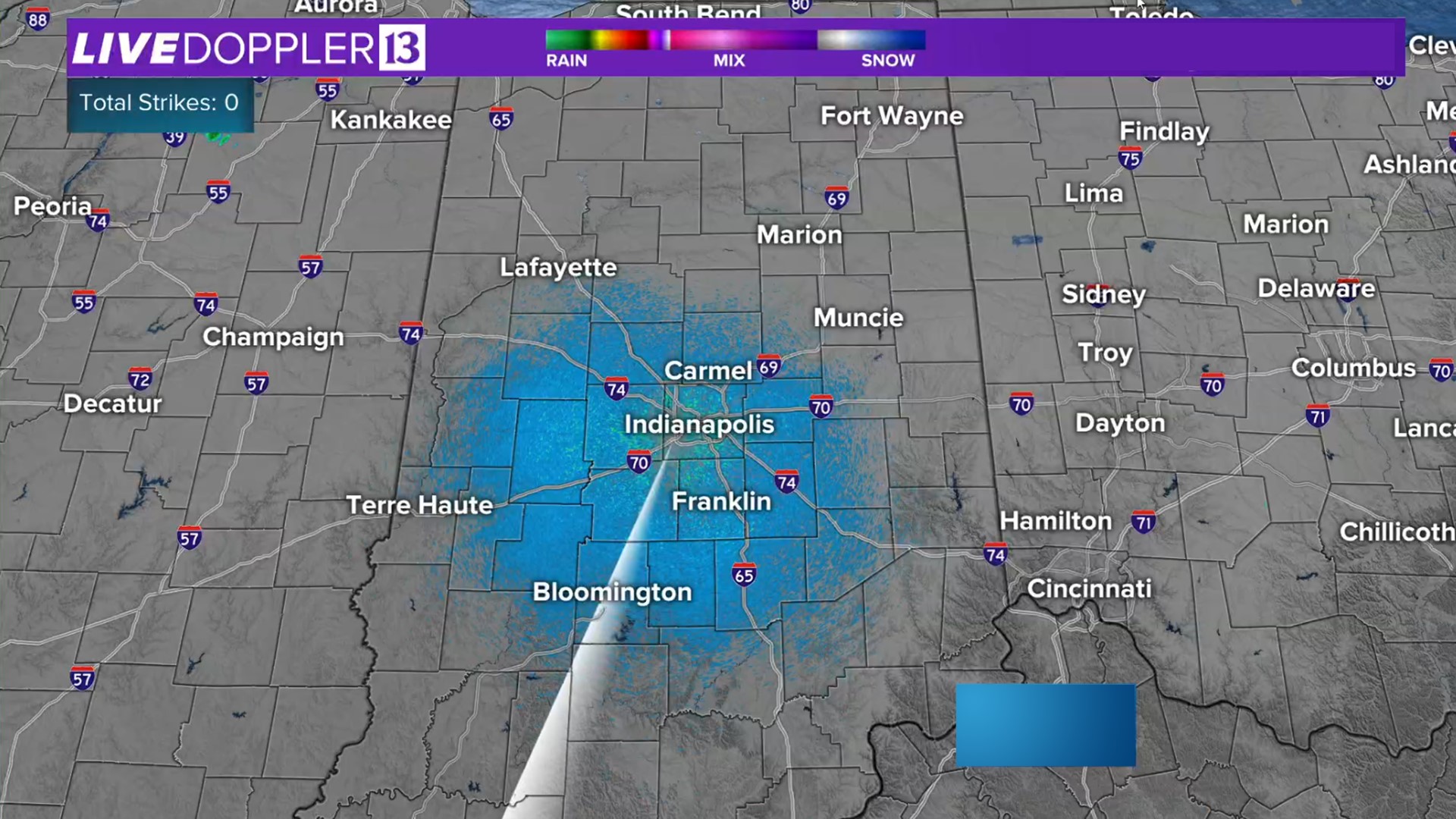This image features a weather map likely used for a nightly news broadcast or a weather app, focusing on the Central Midwest region, including parts of Ohio, Indiana, and Illinois. The top of the image displays a purple banner labeled "Live Doppler 13." Below this banner, a detailed color key ranges from green to purple, indicating different types of precipitation: green for rain, pink and purple for a mix, and bluish-white for snow. The map itself is gray and outlines various counties and cities, such as Peoria, Decatur, Champaign, Lafayette, Fort Wayne, Marion, Muncie, Findlay, Lima, Sydney, Troy, Dayton, Hamilton, and Cincinnati. The central focus is on Indianapolis and its surrounding cities like Carmel, Franklin, and Bloomington, highlighted in blue, indicating snowy conditions. The map also shows major highways such as Route 74, Route 70, and Route 65, with the label "total strike zero" at the bottom, presumably indicating no lightning strikes.